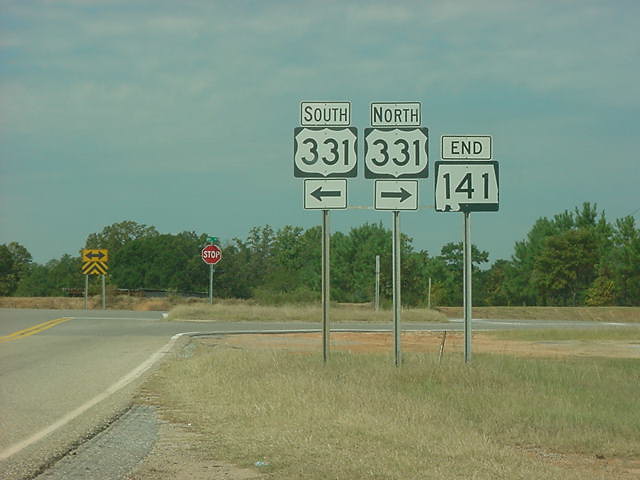Under a vast blue sky adorned with scattered clouds, a vivid scene unfolds. On the left side of the image, a bright yellow road sign stands prominently. To the right of it, a red sign boldly content takes its place. In the background, lush green leaves from towering trees frame the scene, adding a splash of natural beauty against the man-made elements.

The ground is comprised of a gray asphalt road, visibly weathered but clearly marked with yellow lines that run along its center, guiding travelers. In the bottom right corner, patches of dry grass and fields of dirt add a touch of rustic charm to the otherwise orderly setting.

Several signs provide directional information: one informs drivers that they are heading south, while an interstate shield displays "331" to the left, and another sign directs northbound traffic on "331" to the right. Lastly, the red sign declares "End 141," marking the conclusion of a route. This detailed tableau captures the intersection of nature and infrastructure on a clear, sunny day.